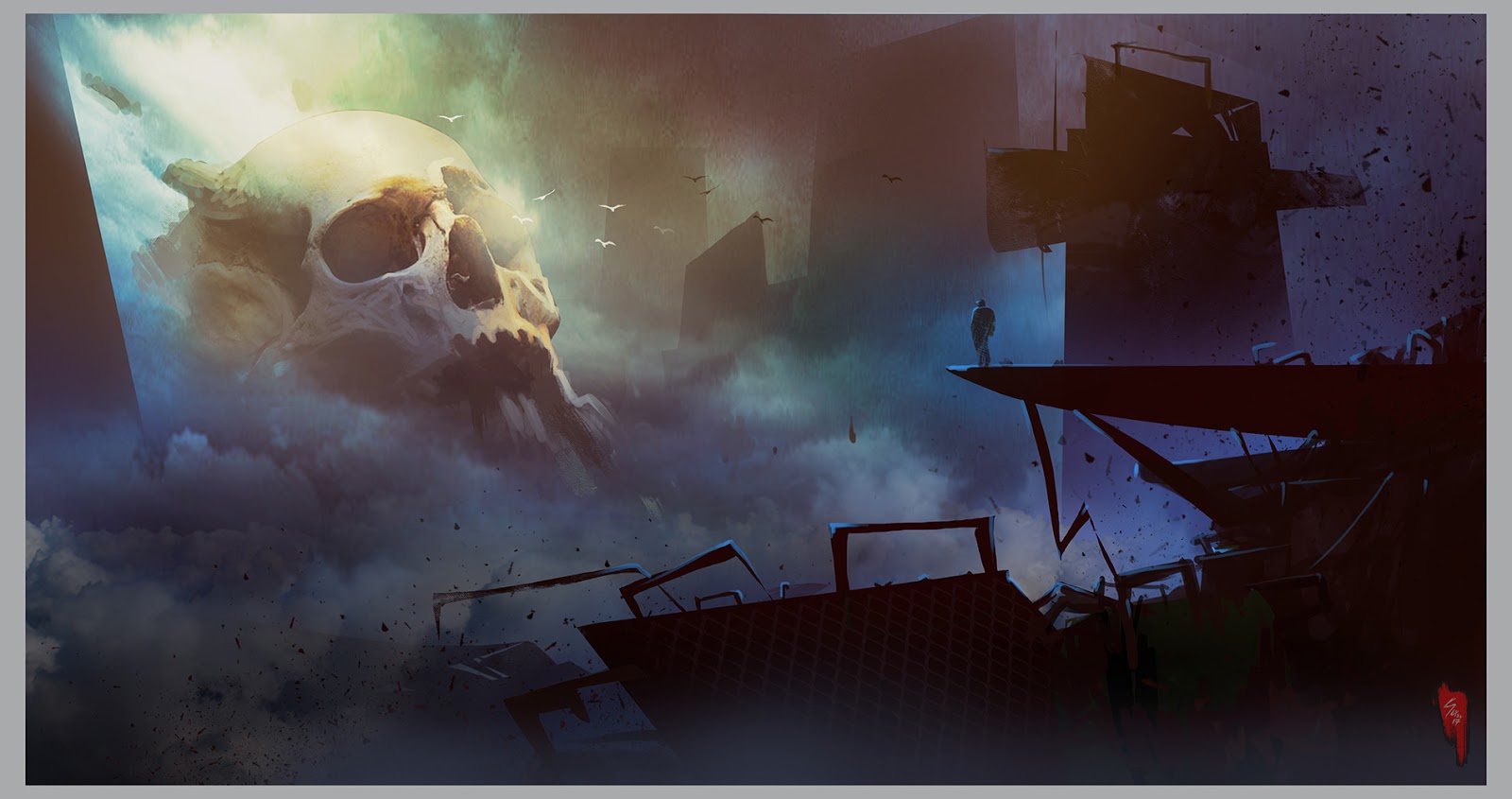The digital artwork depicts a haunting scene in a landscape mode that combines elements of a shipwreck and a destroyed cityscape, all enveloped in a ghostly atmosphere. The left side of the image features a colossal, weathered human skull, partly overgrown with vegetation and surrounded by mist and clouds. Sunlight beams down from the upper left corner, illuminating the skull which has a ghostly white and bone color along with tinges of green and light blue. Birds can be seen flying around the skull, adding to the eerie ambiance.

On the right side of the image, the terrain shifts to a desolate area filled with debris. There are broken buildings, smashed metal, and remnants of ships scattered amidst a landscape of jagged, irregular structures. From the center of this chaotic scene extends a long metal promontory, at the end of which stands a solitary figure gazing towards the skull. The colors on this side are predominantly blacks, reds, and grays, suggesting destruction and decay.

In the bottom right corner, a red splotch of paint with white text—presumably the artist's signature—adds a subtle touch of color and intrigue, though the text is not legible at this resolution. The overall mood of the artwork is somber and enigmatic, combining the ghostly remnants of shipwrecks with the eerie presence of a gigantic skull in a destroyed, foggy landscape.